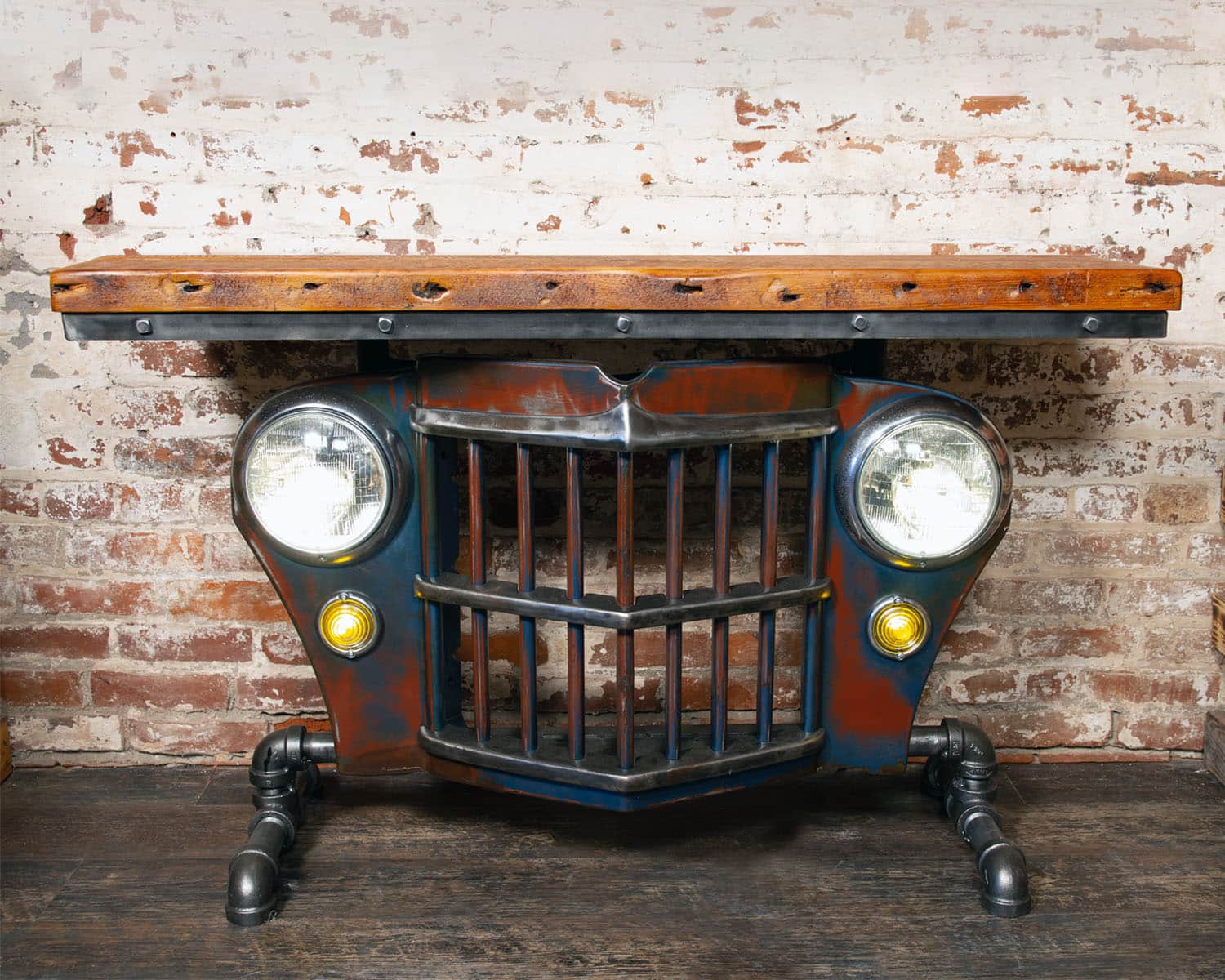Against a rustic, exposed brick backdrop with a weathered wooden floor, this striking upcycled table commands attention. The table is ingeniously crafted from the front grille of a vintage car, featuring a pair of prominent, clear, and silver headlights with smaller yellow lights beneath. The distressed grille, showcasing hues of blue, red, and patches of rust, forms a square rectangular shape that draws the eye. Metal plumbing pipes ingeniously act as the table’s legs, adding a steampunk aesthetic. The centerpiece of the design is the open grille, reminiscent of a prison cell, highlighting the table's industrial charm. Atop this assembly, a flat metal platform supports a reclaimed wooden tabletop, merging seamlessly to create a functional and evocative piece of furniture.